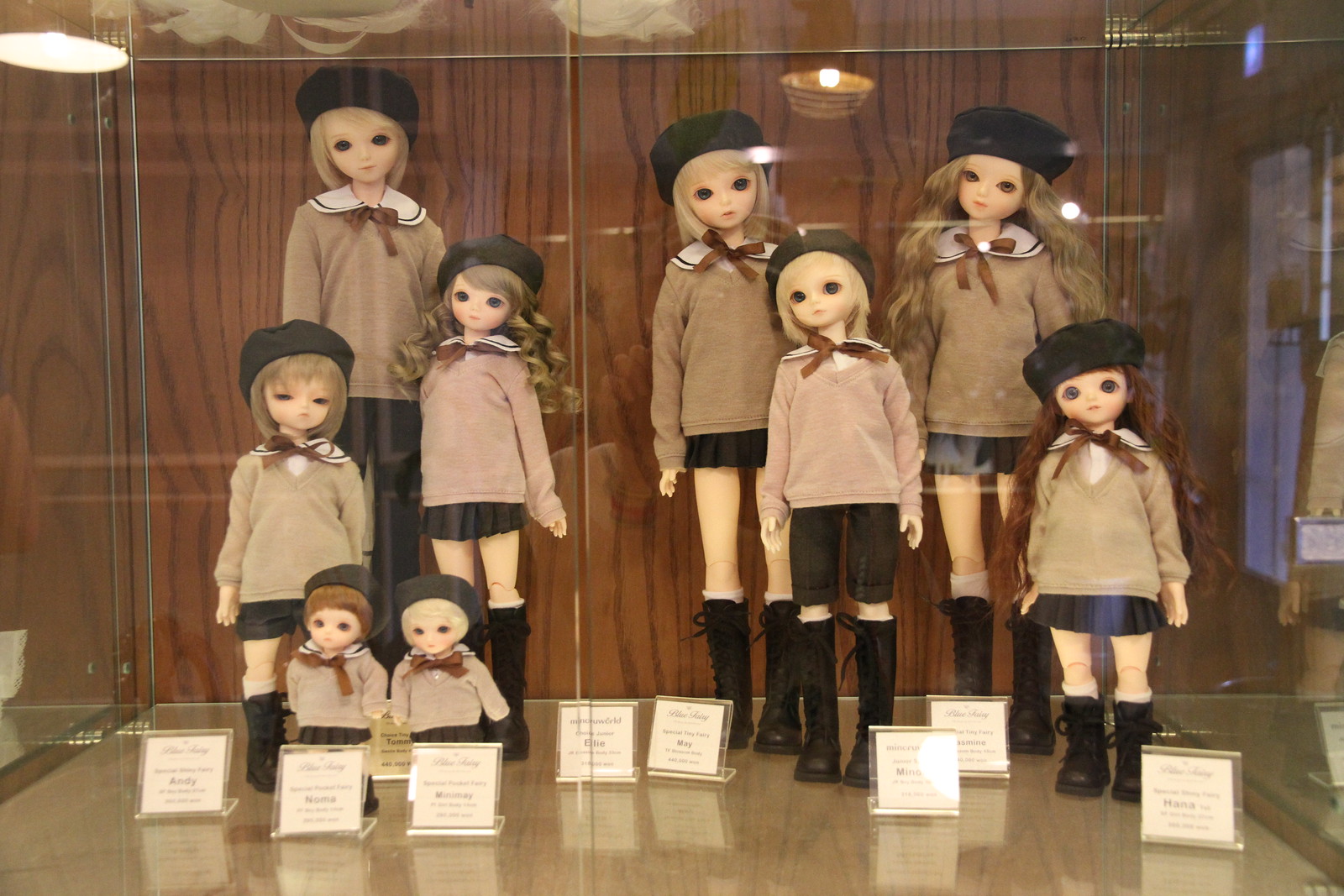This photograph captures a group of porcelain dolls of various sizes, displayed in a glass case with a wooden background and a tan-dark beige floor. The dolls range in size from tall to small, including baby dolls and what appear to be pre-teen or teenage dolls. Each doll has distinct facial features and hairstyles, including blonde and long dark brown hair, and they are topped with berets that resemble military caps.

These dolls are dressed in a variety of school uniform-like outfits, featuring primarily light brown long-sleeve shirts with white collared undershirts adorned with brown bows. Some of the dolls also wear pink or off-pink sweaters, as well as black skirts or shorts paired with knee-high black boots. Each doll has a small white placard with unreadable text in front of it, indicating their individual names or other identifying details. Their upright posture and forward gaze suggest a formal display, and the indoor setting is confirmed by the reflection seen in the top right corner of the image.